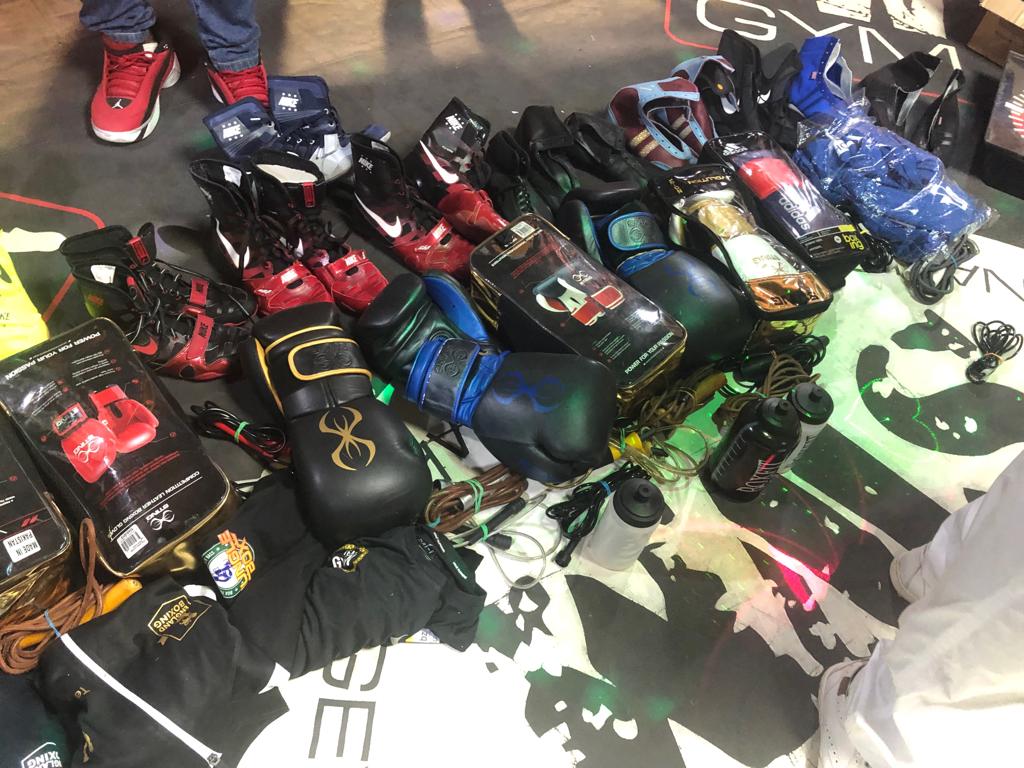This photograph captures a vibrant street stand setup featuring an array of athletic equipment laid out on what appears to be a black and white mat or rug. Dominating the scene are numerous pairs of boxing gloves, around eight, in colors ranging from black to red to blue, some still encased in packaging. Alongside the gloves, various types of shoes can be observed, predominantly red and black, with one pair boasting a striking combination of blue, red, and gold. Interspersed among them are additional athletic items including black shirts or tops with logos, shirts inside a glass case, three water bottles with black caps, and a plethora of wires and cables mixing with the equipment. The scene is lit by outdoor sunlight, casting a natural shine over the objects. Two people are partly visible; one in the background wearing Air Jordans, seemingly looking down at the display, and another whose red shoes and the lower part of blue jeans peek into the frame. On the floor, there's black font writing against a white background, but much of it is chipped away, revealing patches of white beneath. This vivid assortment creates an intriguing display that hints at a casual, makeshift marketplace ambiance.